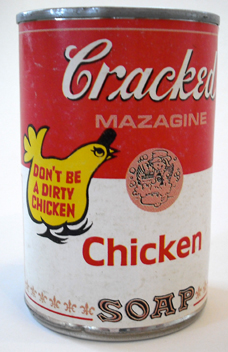This image features a can of soup set against a light gray background, closely resembling a classic Campbell’s soup can but with key differences. The metal can is designed with a metal ring at both the top and bottom. The upper section of the label is red, adorned with the word "cracked" in bold white letters, followed by the word "magazine" in gray letters. A small circle on the label displays pinkish-brown spots for added detail. A prominent yellow chicken is catching attention, emblazoned with the phrase "Don't be a dirty chicken" in red letters. The lower part of the label is white, featuring the word "chicken" in red, followed by "soap" in a mix of gold and black fonts, indicating the can contains a playful or satirical product rather than actual soup.